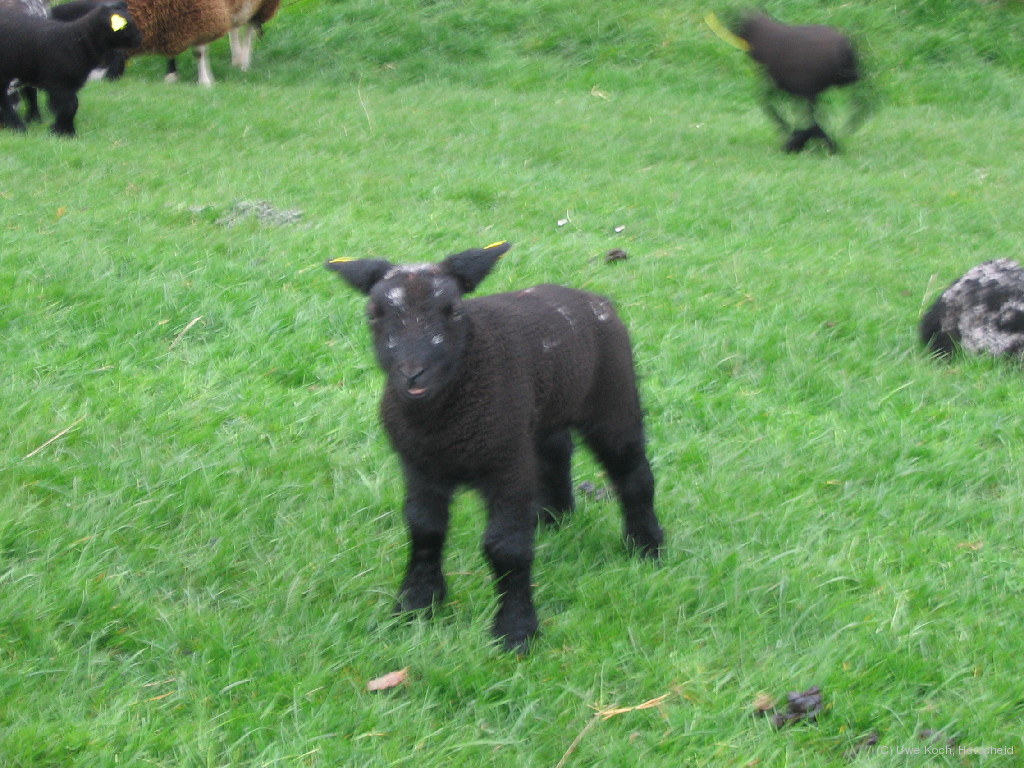This is a photo of a small, black baby sheep standing in a lush, green field. The sheep has pointed ears, an angular face, and a furry body supported by four large legs. Despite the slight blurriness of the image, you can discern several other animals in the background. There is a brown sheep in the upper left corner with its head not fully visible, and another black sheep appears to be running at full speed in the upper right background. The field is dotted with a few blackish-grayish stones, with one particularly noticeable in the bottom right and another towards the center right. Near the top left of the image, just above the baby sheep's head, there seems to be a hint of flowers, though they are hard to identify due to the photo's blur. Overall, the image captures a serene scene of young sheep scattered across a vibrant grassy landscape.